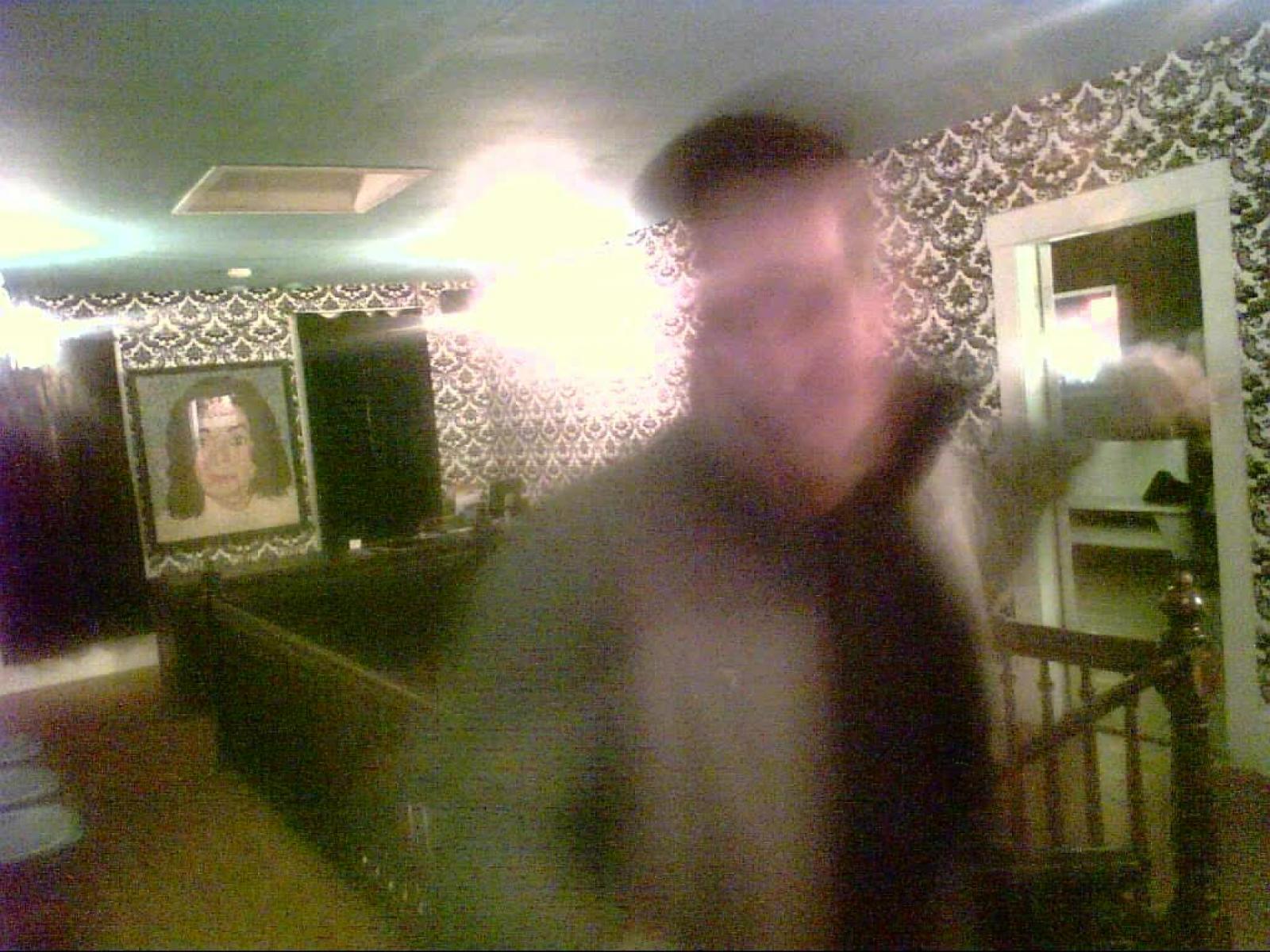This indoor, slightly blurry color photograph appears to be taken on the second story of a home, capturing a man standing in front of a stairwell with brown carpet and rails. The man, who has short brown hair, is dressed in a whitish-gray jacket over a green or black shirt and is making a fist with one hand pulled back. Despite the blur, it's clear he has just ascended the steps. The background showcases distinctive white and black diamond-patterned wallpaper and a doorway to the right that leads to another room. Noteworthy is the prominently framed portrait resembling Michael Jackson with black hair, wearing a white shirt, positioned on the furthest wall. The ceiling above features a white vent and emits a bright, shiny light.